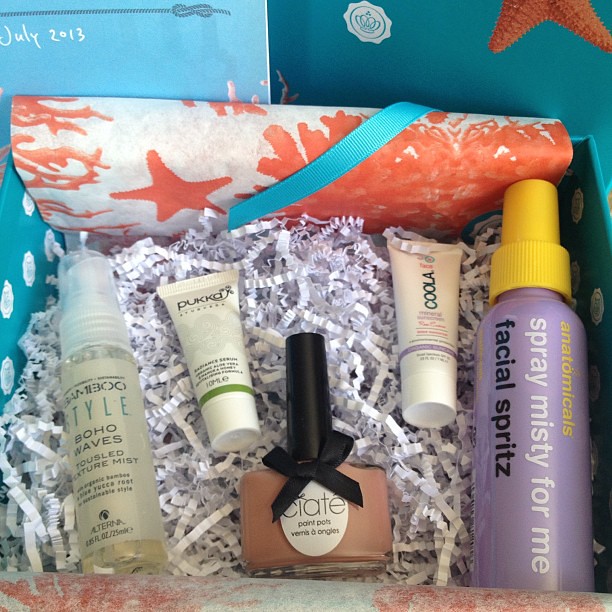This color photograph captures a top-down view inside a blue gift box adorned with undersea starfish and coral designs, marked with the date "July 2013" in white handwriting script. The box is lined with shredded white paper. In the center lies a gift-wrapped package in bright orange and white with undersea motifs, tied with an aqua blue ribbon. Arranged inside the box are five beauty products. On the far left is a transparent spray bottle labeled "Bamboo Style Boho Waves" with a clear cap. Next to it is a small white bottle with the label "Pukka" and a plant logo indicating it holds 10 ml. In the center is a short clear bottle of brown nail varnish branded "Siete," tied with a black ribbon and topped with a tall black cap. Immediately to its right is a small white square tube labeled "Koola." On the far right is a tall lavender spray bottle with a yellow cap labeled "Anatomicals Spray Misty for Me Facial Spritz." This tightly composed image showcases a curated selection of beauty products, highlighting textures, colors, and branding details.